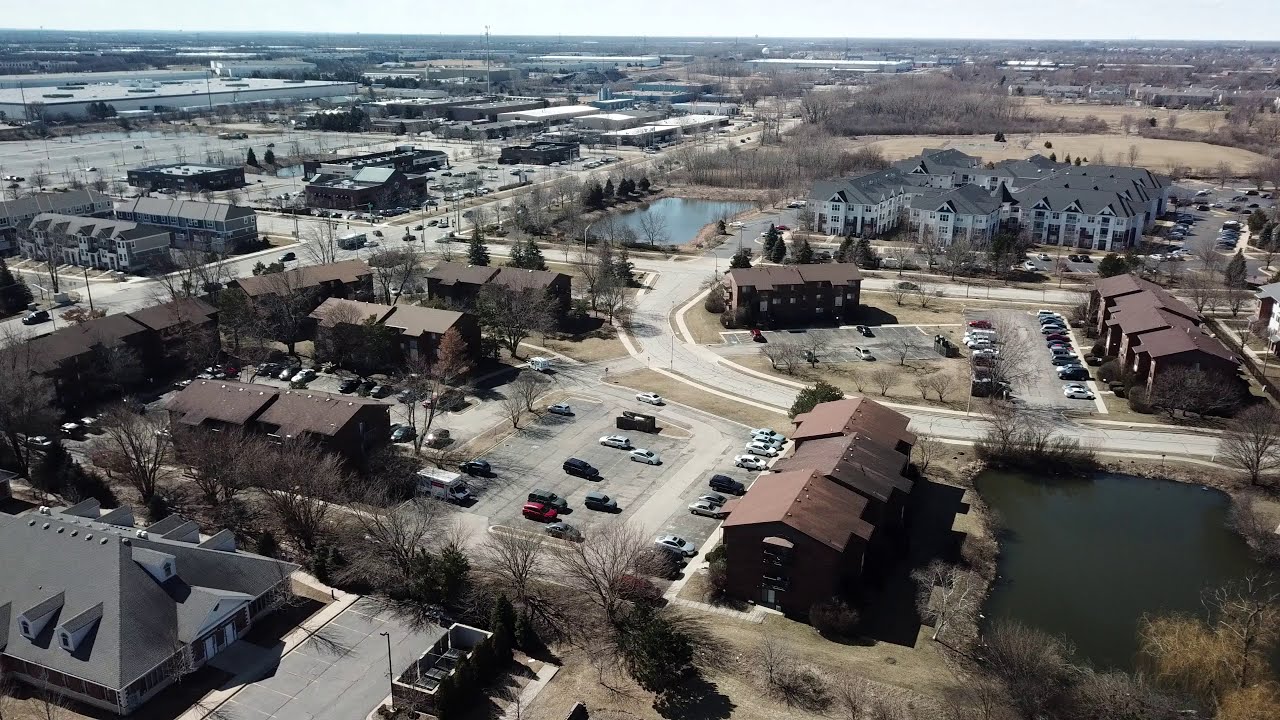This aerial photograph captures the suburban edge of a town, showcasing a variety of two- to three-story townhomes and condominiums with brown roofs. The buildings are closely packed, and a noticeable feature is a small pond, dark in appearance, located at the bottom right of the image. The pond is encircled by barren trees and dirt patches, hinting at a possible late autumn or winter season as the trees lack leaves. Numerous parking lots dotted with cars, vans, and pickup trucks are scattered throughout the scene.

In the lower left, there's a large, steep-roofed building with dormers that could be a business, perhaps a shop, conference center, or even a funeral home. Additional structures include taller apartment buildings and commercial buildings in the background, with varying colors of black, white, and gray. The upper left features a vast warehouse, evoking the style of a Sam's Club rather than an Amazon distribution center, and to the upper right, there’s a green, grassy area with some trees, which may be a park. Roads crisscross the landscape, connecting parking lots with the wider town infrastructure, including a major roadway from mid-left to top-right. The sky forms a thin, hazy, whitish-blue band along the horizon, adding to the expansive view of this suburban-town edge from a high vantage point.